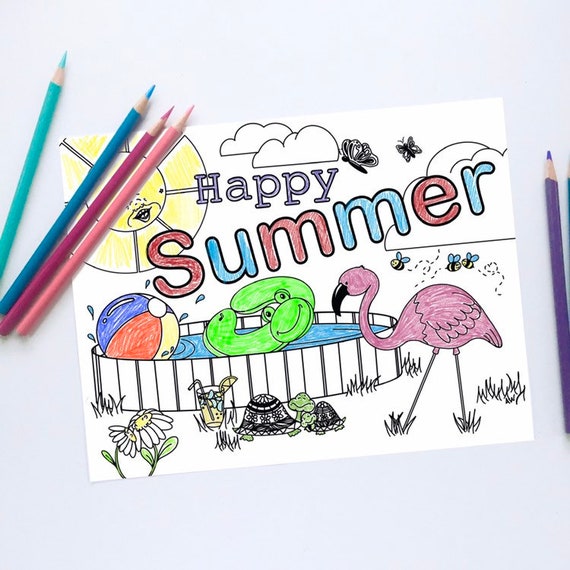A vibrant coloring page lies on a white to light blue table, adorned with a variety of colored pencils including pink, dark pink, dark blue, cyan blue, and purple. At the top of the page, the words "Happy Summer" are prominently displayed, with "Happy" colored in purple and "Summer" colored in alternating red and blue letters. Surrounding this cheerful message are whimsical details: a smiling sun with eyes and a nose in the top left corner, fluffy clouds in the upper middle, and butterflies fluttering near the text. A flamingo stands tall to the right, while bees buzz nearby.

In the middle section, there is an above-ground swimming pool, white and mostly uncolored, featuring a green frog floatie and a red, white, and blue beach ball. To the bottom right of the pool, a big turtle and a small turtle bask next to a glass of lemonade filled with ice and topped with a straw and lemon slice. On the bottom left, some dandelions and white daisies with yellow centers add a touch of nature.

The coloring is partially completed, with the pink, dark pink, dark blue, cyan blue, and purple pencils strategically placed around the paper, suggesting a child’s ongoing delightful summer project.